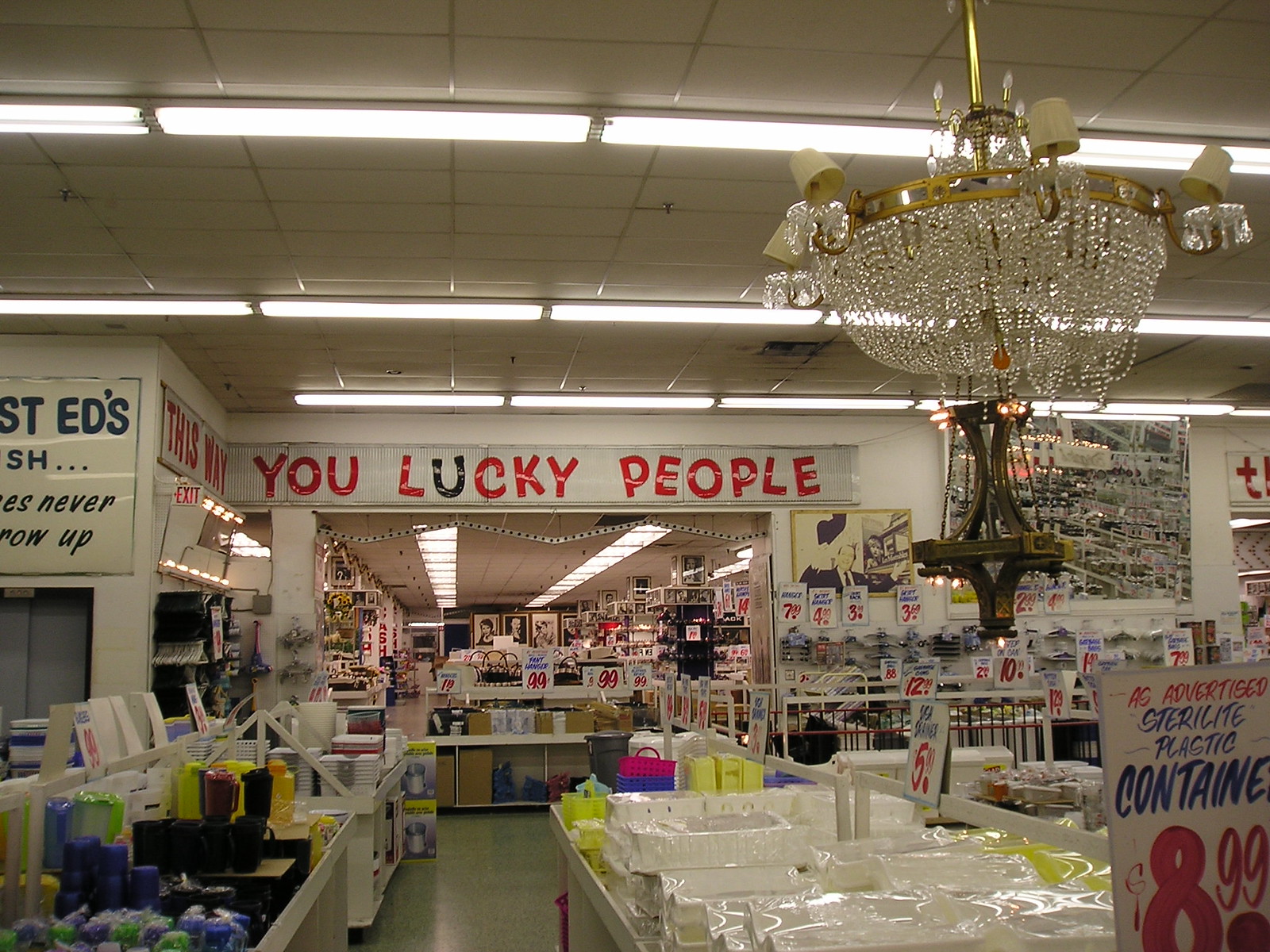The image depicts an interior of a retail store. At the top right corner, a crystal chandelier adorned with tiny lampshades catches the eye. It is beautifully illuminated, adding a touch of elegance to the space. Along the ceiling, three rows of bright, horizontal ceiling lights stretch from the front to the back of the image, ensuring the store is well-lit.

At the back of the store, a prominent sign reads "You lucky people" with all letters in red except for a black "U" in the word "lucky." This quirky detail adds a playful element to the signage. To the left of this main sign, there is a partial sign in white with blue text. The visible text reads "Ed's" followed by "ST" to the left, and beneath it, the letters "SH...ES," the word "never," and on the last line, "ROW up."

The store is bustling with various items for sale. White signs with red text stating "As Advertised" and blue descriptions of items are scattered throughout. In the bottom right corner of the image, there is a blue Sterilite plastic container with a red price tag reading $8.99. Numerous other white Sterilite plastic containers are also visible, hinting at a sale. The background showcases various framed pictures and artworks available for purchase, both on display and hanging on the walls, adding to the store's eclectic merchandise.

Overall, the combination of elegant lighting, playful signage, and a myriad of items for sale creates a lively and inviting shopping atmosphere.